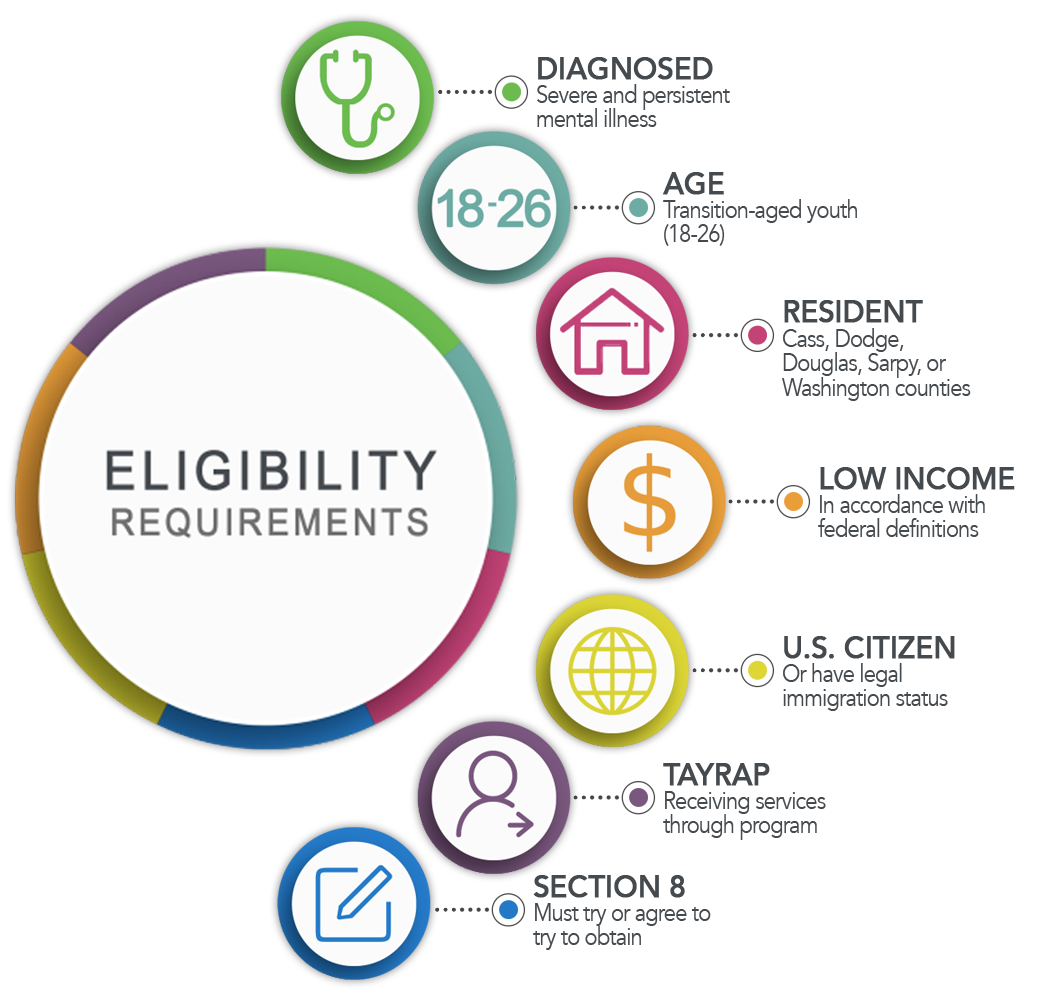The image is a detailed, multi-colored informational graphic set against a white background. Central to the design is a large white circle bordered by segments in vibrant colors: purple, green, blue, pink, dark blue, yellow, and orange. This central circle contains the text "Eligibility Requirements" in black. Surrounding the right half of this main circle are seven smaller circles, each of which is color-coded to match one of the segments of the larger circle's border. These smaller circles and their corresponding icons and titles represent different eligibility criteria: 

- **Diagnosed** (stethoscope icon, purple)
- **Age** (18 to 26 icon, green)
- **Resident** (house icon, blue)
- **Low Income** (dollar sign icon, pink)
- **U.S. Citizen** (world sign icon, dark blue)
- **TARAP** (outline of a head and a belly with arrow icon, yellow)
- **Section 8** (notepad with pen icon, orange)

Each smaller circle has black text next to it, offering brief descriptions of the corresponding eligibility requirement. The orderly arrangement and clear, color-coded design make it easy to discern the detailed eligibility criteria at a glance.